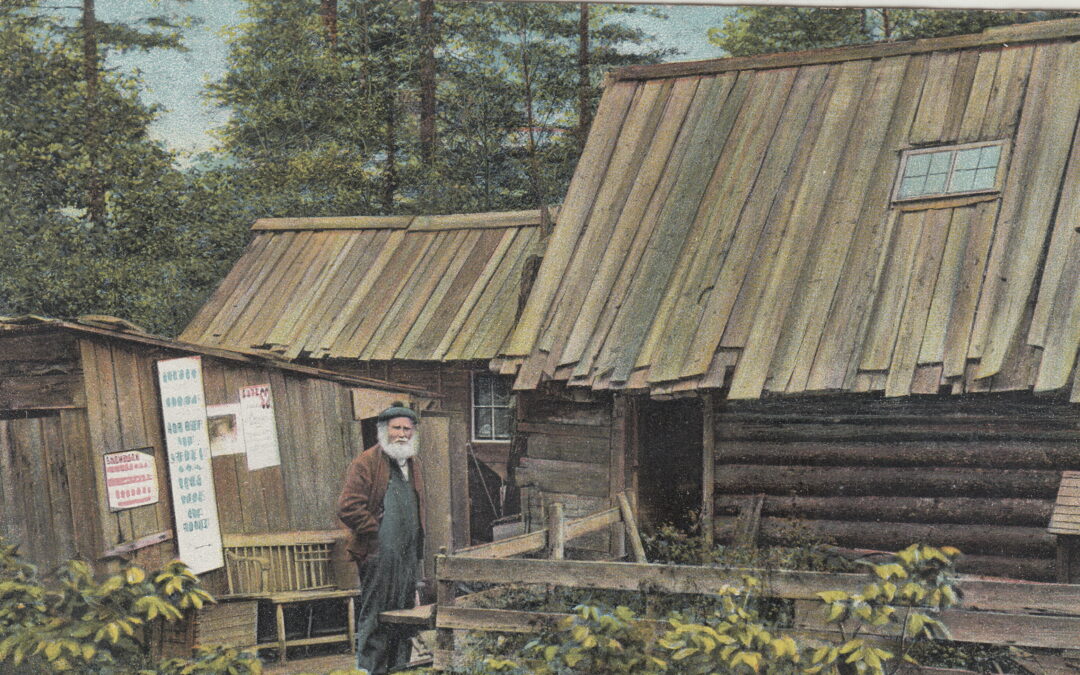The image captures a 1920s-30s setting in the Appalachian Mountains, showcasing a rustic scene with a dense forest backdrop. Dominating the foreground is an old cabin made from individual wood slats, complemented by a handmade wooden bench and surrounded by verdant plants. Adjacent to this cabin, there are two additional structures, one appearing to be an outhouse and the other a shed. The buildings feature multiple windows, with the cabin roof housing two, and several illegible signs adorn the shed's side.

A notable figure stands central in this scene: an elderly Caucasian man with a long, white beard, exhibiting a somber expression. He wears a brown hat, a brown jacket, and bib overalls, his hands relaxed in his pockets. The color palette of the painting includes vibrant greens from the background trees and foliage, as well as touches of yellow, brown, blue, and white, suggesting a digitally captured image of a painting.